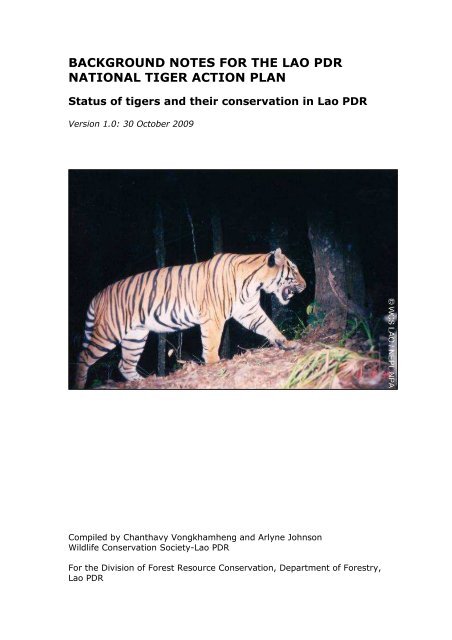The image features a news article titled "Background Notes for the Lao PDR National Tiger Action Plan: Status of Tigers and Their Conservation, Lao PDR, Version 1.0, 30 October 2009." The focal point of the article is a vivid nighttime photograph of a tiger, captured in a dark forest. The tiger, illuminated by a flash, showcases its striking orange and black stripes as it appears to be roaring or growling from a profiled perspective, possibly sensing danger. The black background accentuates the tiger's majestic and foreboding presence as it prowls the forest floor. The compilation of the article is credited to Chanthavy Vankhamhang and Arlene Johnson from the Wildlife Conservation Society-Lao PDR, prepared for the Division of Forest Resource Conservation, Department of Forestry, Lao PDR.